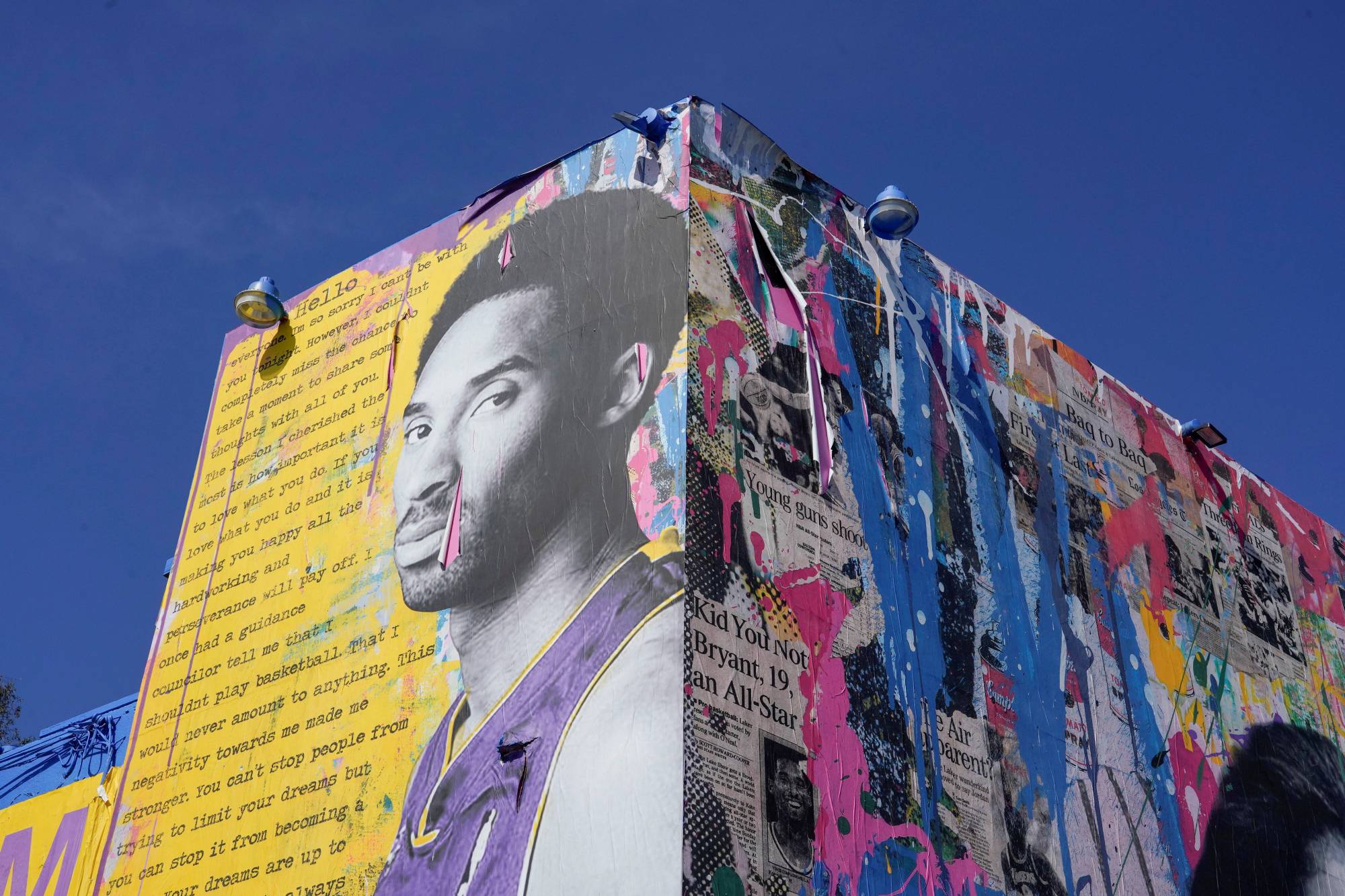This detailed full-color photograph, captured outdoors on a clear, cloudless day using natural light, showcases an intricate mural of the late basketball player Kobe Bryant. Positioned at the corner of a building, the square image focuses on the building's front and left side walls. The mural is highly realistic, depicting Kobe Bryant primarily in black and white, wearing a striking purple jersey. His profile, with head and eyes turned towards the viewer, forms a central part of the left wall. Above him, a yellow section features a typewritten quote, attributed to Bryant, offering inspiring words about hard work and perseverance, although some text is partially obscured.

On the right side, the mural transitions into a vibrant collage of graffiti, dripping paint in blue, pink, and yellow hues, overlaying various newspaper headlines and articles about Kobe Bryant. The dynamic mix of colors and textures contrasts with the clear blue sky that serves as the mural's serene backdrop. Three overhead lights crown the mural, illuminating both its artistic and commemorative essence.